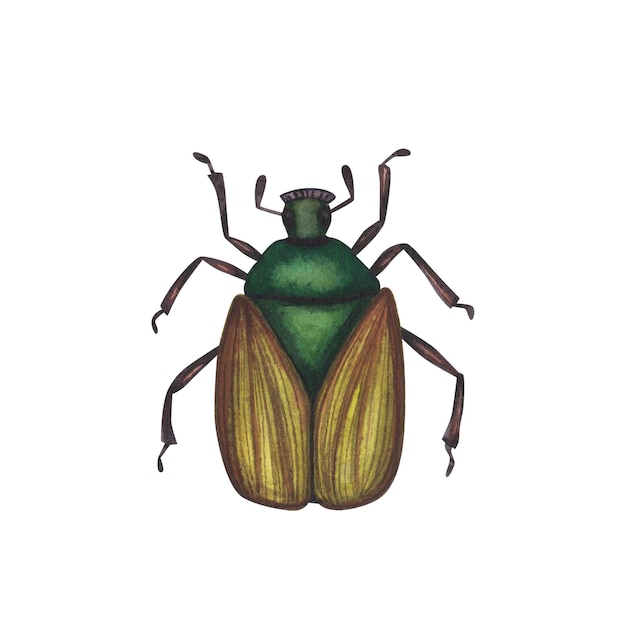The image is a detailed, colorful drawing of a beetle set against a plain white background. The beetle has a bright green thorax and head, adorned with two brown antennae of the same shade as its six spindly, elbow-jointed legs. The wings, tucked neatly against its body, exhibit streaks of brown and yellow, contributing to the intricate shading and texture that suggest a high degree of artistry, possibly achieved with colored pencils or art crayons. Its eyes are darker blue and inset, adding to the lifelike quality of the drawing. Additionally, there is a small, crown-like marking on top of the beetle's head, and a fan-like appendage near its mouth, presumably for sensory perception.